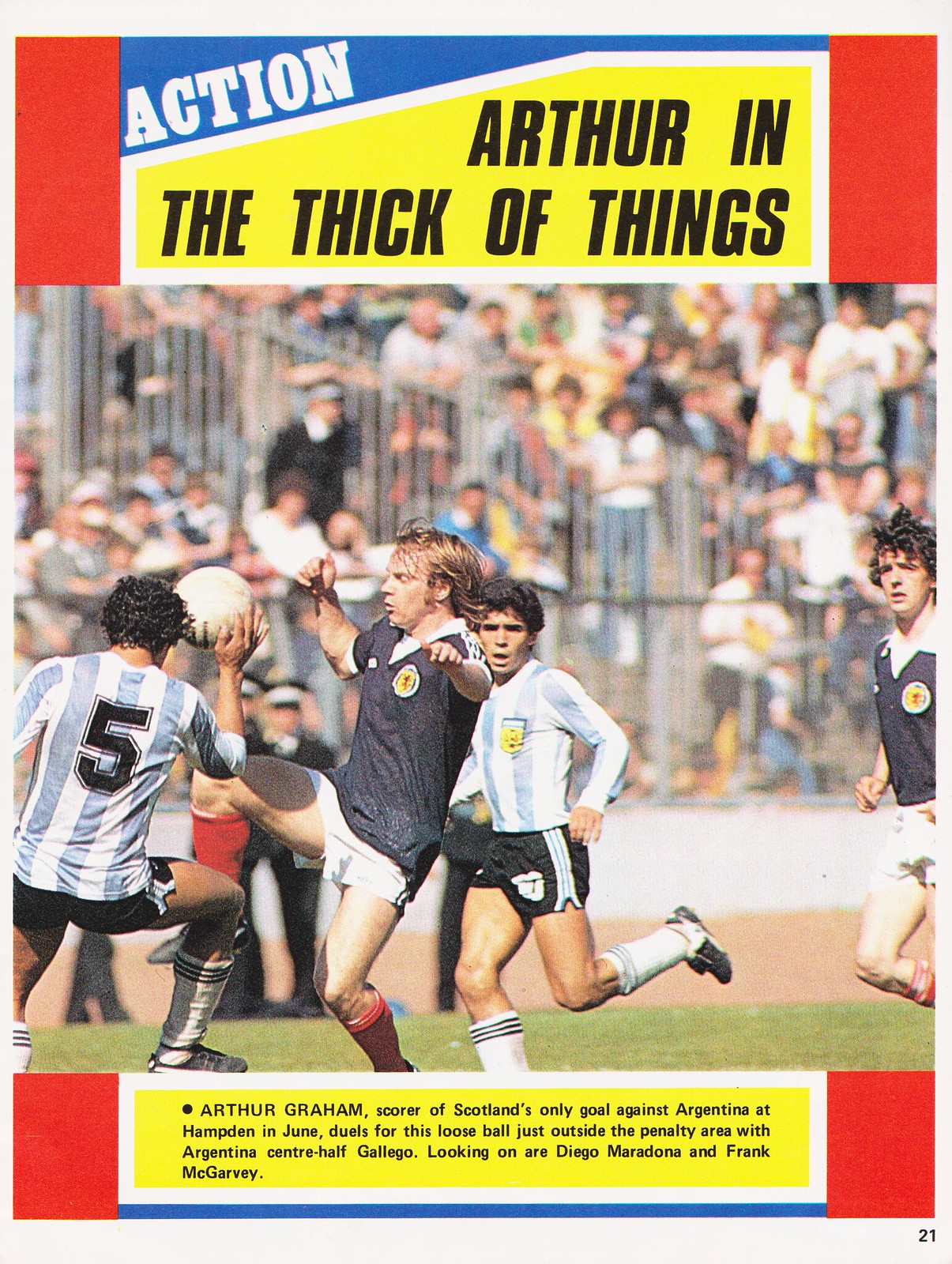The image is the cover of a magazine featuring a detailed depiction of a soccer match. At the very top, set against a blue background, the word "ACTION" appears in white slanted print. Beneath that, on a yellow background with red borders on each side, is the headline "ARTHUR IN THE THICK OF THINGS" in black print. The central part of the cover showcases a dynamic soccer scene with four to five players in action. On the left is a player wearing a blue and white vertically striped jersey with the number 5 on his back and black shorts, likely the goalie. To his right, an opponent in a dark jersey and white shorts extends his right leg towards the ball. Behind him, another player in a blue and white striped shirt and black shorts is running with his left leg in the air, followed by another opposing player in a dark jersey and white shorts. The players are positioned in front of a packed crowd of spectators, visible through silver gates, creating a vibrant backdrop. At the bottom of the image, on a yellow background with red borders on either side, the text reads: "ARTHUR GRAHAM, scorer of Scotland's only goal against Argentina at Hampden in June, duels for this loose ball just outside the penalty area with Argentina center-half Gallego. Looking on are Diego Maradona and Frank McGarvey." The field is green, capturing the vivid scene of an outdoor soccer match.